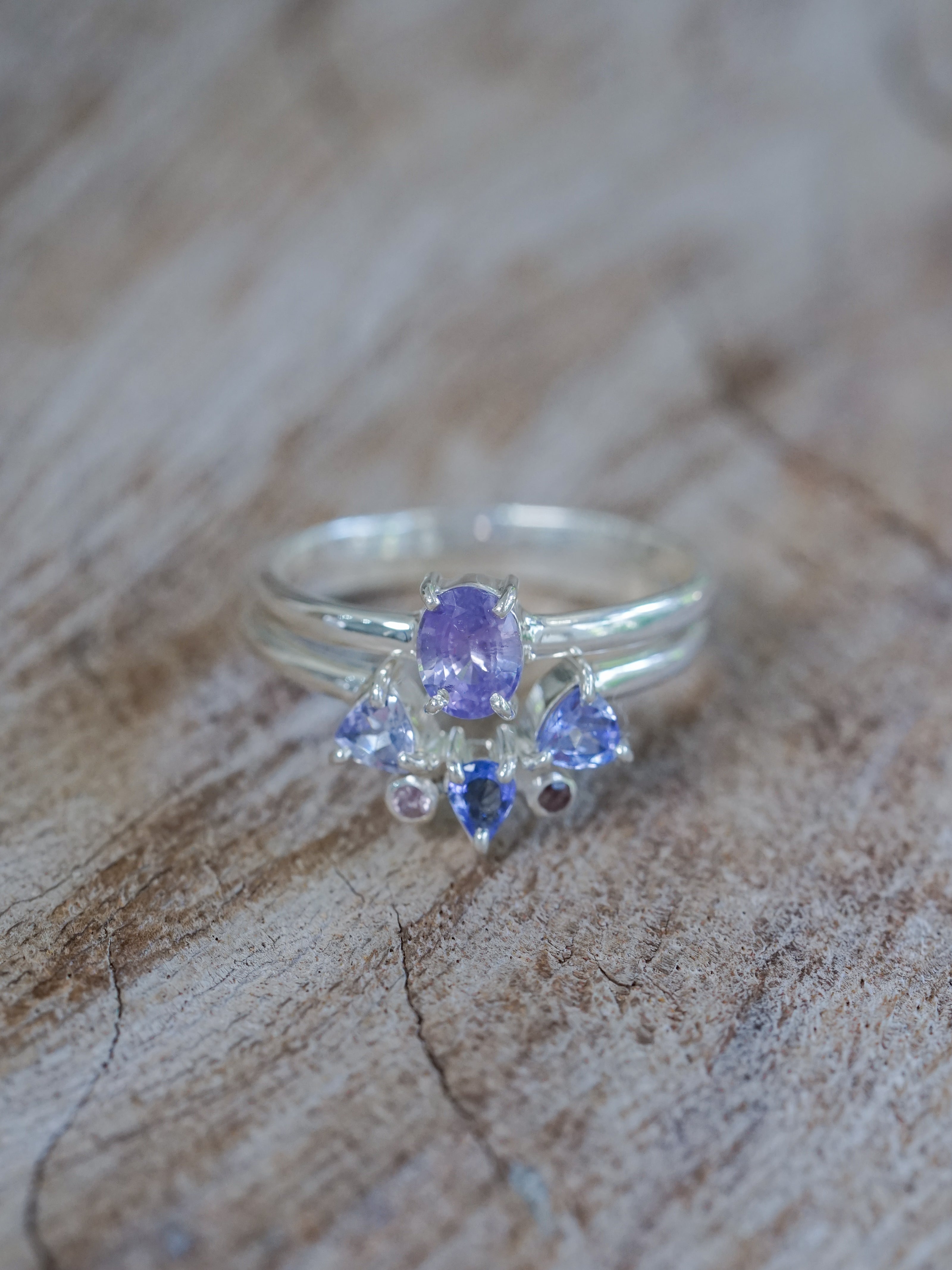This is a detailed close-up image of a silver ring with a double band. The ring features a variety of gemstones. At the top, the largest stone is an oval-shaped gem of a purple-blue hue, held in place by white claw-like prongs. Beneath this prominent gemstone is a dark blue tear-drop shaped gem that appears to have black inclusions or shadows in its center. Flanking this central gem are two diamond-shaped dark blue stones, while to the sides, there are small round gems—one light blue and one sapphire blue. Additionally, there are two smaller circle gems: one on the left, which is a whitish-purple color, and one on the right, which is black. These gemstones are elegantly set in a design that resembles a flower pattern. The ring is resting on a surface that appears to be either a piece of textured wood or a fabric with a wood-like pattern, characterized by its varying shades of brown and cream, as well as visible grain and cracks. The background of the image is blurred, making the detailed design of the ring the focal point.